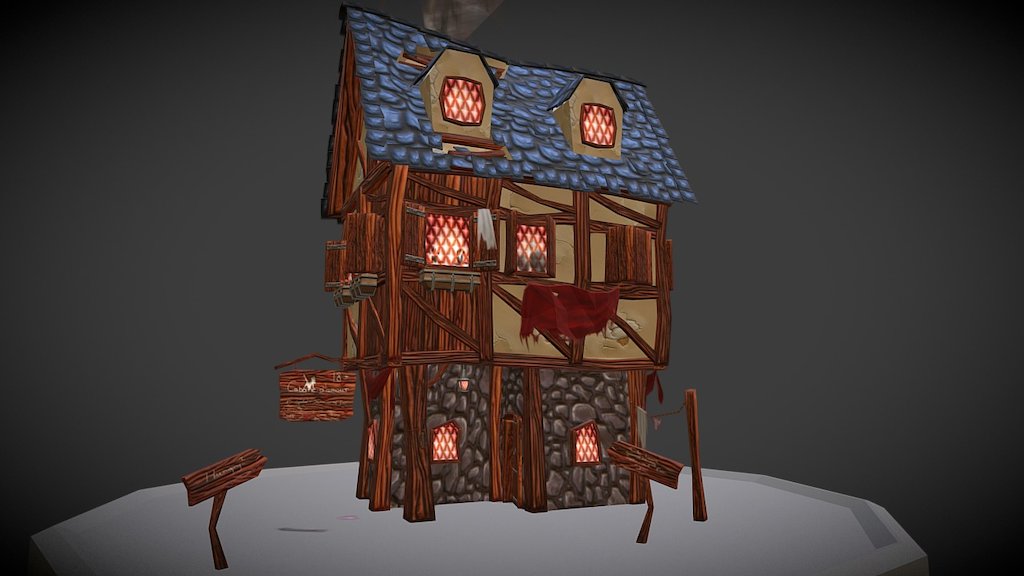This image appears to be a computer-generated 3D rendering of a rickety, three-story cottage situated on a lighter grey ground with a darker grey background. The bottom of the house is constructed from stone, while the upper floors feature wooden framing and a tan exterior, with shingles covering the blue roof. The cottage features numerous windows: the ground floor has several windows and a door, all seemingly illuminated by candlelight from within. The second floor has three windows, one of which has shutters closed, and the roof has two dormer windows with lattice designs. Additionally, a red flag or cloth hangs outside the building.

The front of the house showcases two wooden signposts with arrows pointing towards the entrance, suggesting some form of invitation or direction. Although the signs' text is indistinct, one appears to inquire if one is "hungry," implying it might be an eatery or restaurant. An additional sign hangs from the left side of the building, further promoting what may be a rustic dining establishment. The entire scene lacks neighboring structures, heightening the isolated, standalone nature of the cottage.